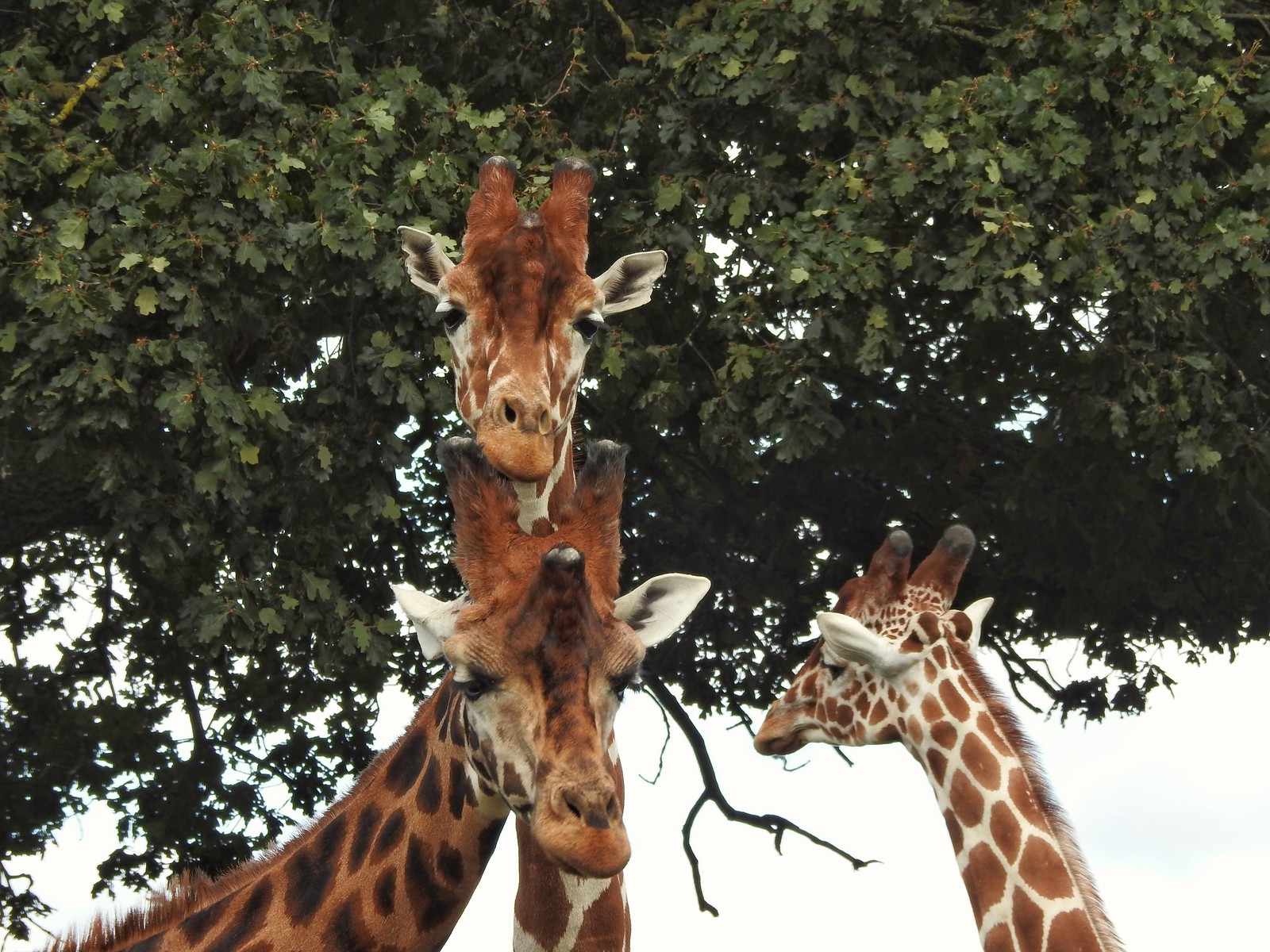This is a detailed photograph capturing three giraffes from their long necks up to their heads, set against a cloudy sky with foliage from a large tree stretching across the top of the frame. The image composition suggests an upward camera angle, giving prominence to the giraffe heads against the backdrop. The giraffe on the right side of the frame has an orange coat with dark brown spots and exhibits a three-quarter profile, focusing on the tree leaves above. The other two giraffes, positioned on the left, are predominantly white with brown spots. The larger giraffe in the foreground, at the bottom left, has its head slightly lowered and its eyes partly closed, exuding a serene, almost sleepy demeanor. Above and entwined with the larger giraffe's horns is a slightly smaller giraffe, facing directly towards the camera with an equally calm expression. All the giraffes feature long ears and distinctive protrusions on their heads, characterized by black-tipped "horns" or ossicones. The intricate pattern of their spots and the tranquil backdrop of the sky and leaves combine to create a captivating and serene wildlife portrait.